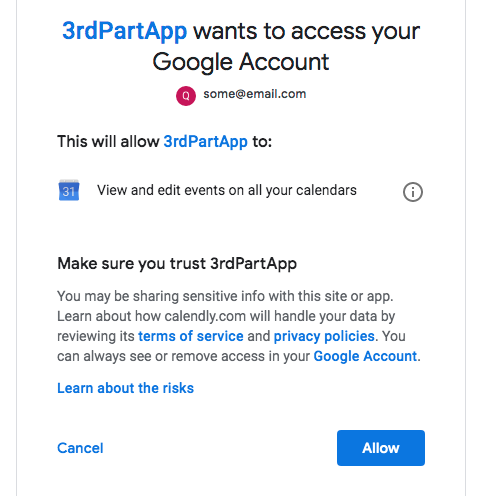Homepage of a Google Account Permission Request for a Third-Party App:

The page features a minimalistic design with a white background and thin gray borders on the left and right sides. At the top of the page, roughly an inch from the left edge, the text "Third-party app" appears in blue, followed by "wants to access" in black, and then "Google account" beneath it. Below this, a red circle with a white "Q" inside it displays an email address (some-email@example.com) in small black text.

On the left side, aligned under the word "third," there is the black text "This will allow," followed by "third-party app" in blue. Below this statement, a blue square with a white "31" is displayed, accompanied by the small black text "view and edit events on all your calendars" and an informational icon represented by a small circle with an "i" in it.

Approximately an inch down, a black warning text reads, "Make sure you trust third-party app" (with "third-party app" corrected from "third-part app"). Further down, a paragraph appears, consisting of four lines detailing terms and services. It states: "You may be sharing sensitive info with this site or app." The next line continues, "Learn about how calendly.com will handle your data by," followed by "reviewing its" in blue. The paragraph ends with "terms of service" in blue, followed by "privacy policies." The final line states, "You can always see or remove access in your Google account," referring to "Google account" in blue, followed by a space and "learn about the risks."

At the bottom left corner of the page, the option to "Cancel" appears, while the bottom right corner features a prominent blue button with the word "Allow" in centered, bold white text.